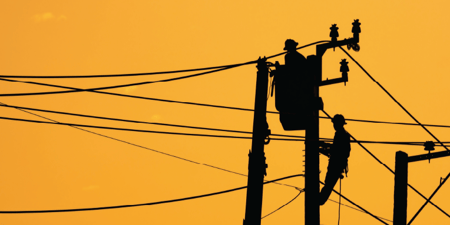The image captures an outdoor scene featuring a vivid gradient sky transitioning from a mustard yellow to a deep orange, suggesting either sunset or sunrise. The background is speckled with a tiny cloud in the upper left corner. Dominating the scene are the black silhouettes of telephone wires and poles, with lines stretching horizontally and diagonally, some curving slightly downward. Two workers, clad in hard hats, are seen silhouetted against the sky: one is standing on a pole, attached by a rope, while the other is elevated higher in a crane-lifted bucket. Additional poles and wires populate the lower right corner, enhancing the intricate web of crossings in the composition.